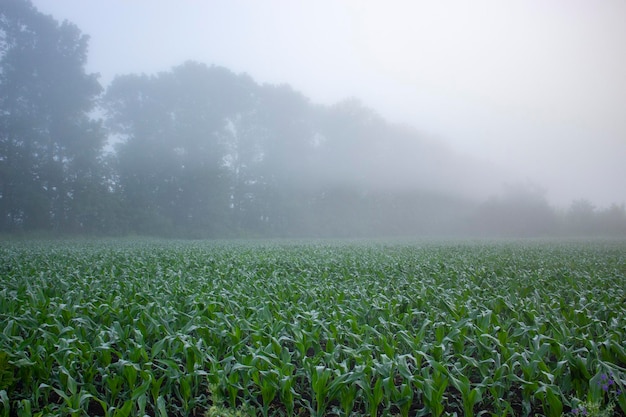The image depicts a foggy, daytime scene of a partially organized, yet cluttered, green field, likely a cornfield on a human farm. The corn stalks are only a couple of feet tall, far from ready for harvest, and are enveloped by a thick layer of fog that dominates the top half of the image, while the bottom half is clearer. In the background, partially obscured by the haze, stands a row of very tall trees, possibly 30 feet high or taller, creating a natural barrier. The sky is overcast and entirely cloud-covered, casting a grayish tone over the scene, though the brightness suggests it is daytime. To the left, the trees appear taller, reducing in height and density as they stretch to the right, indicating a larger forested area surrounding the field.